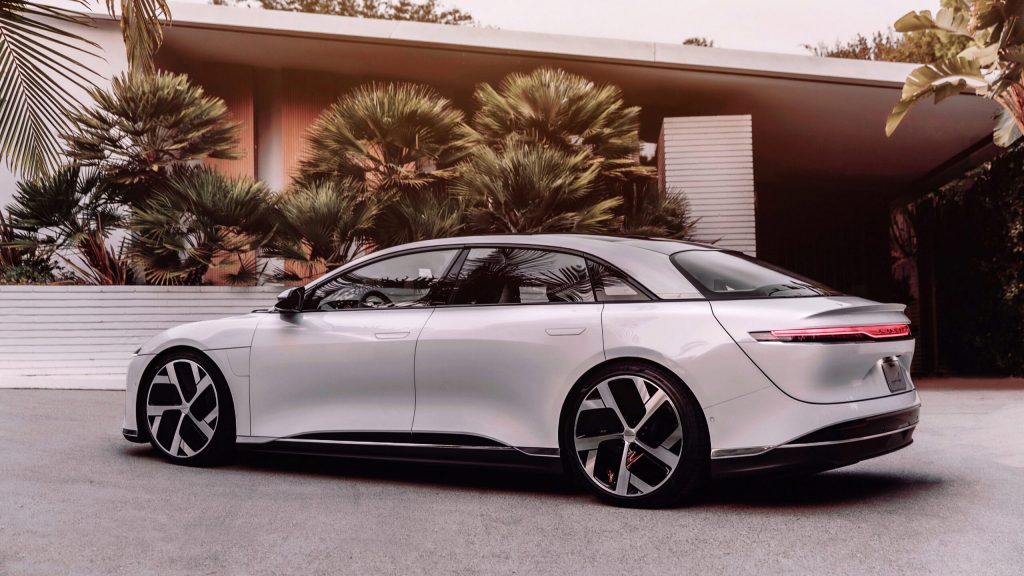The image depicts a sleek, silver four-door vehicle parked on a light gray concrete driveway in front of a modern, well-maintained house. The car, which exudes a sporty and high-tech aura, features a distinctive long red light strip along the back. The surrounding environment suggests a warm, possibly Californian, location with several palm trees and tropical foliage accenting the scene. The house itself has a sophisticated appearance with a mixture of materials: white brick, corrugated metal siding, and a flat roof with white trim. A notable feature is an orange curtain visible through a window behind the trees. The overall composition of the image, with its warm overlay, gives it a polished, promotional quality.